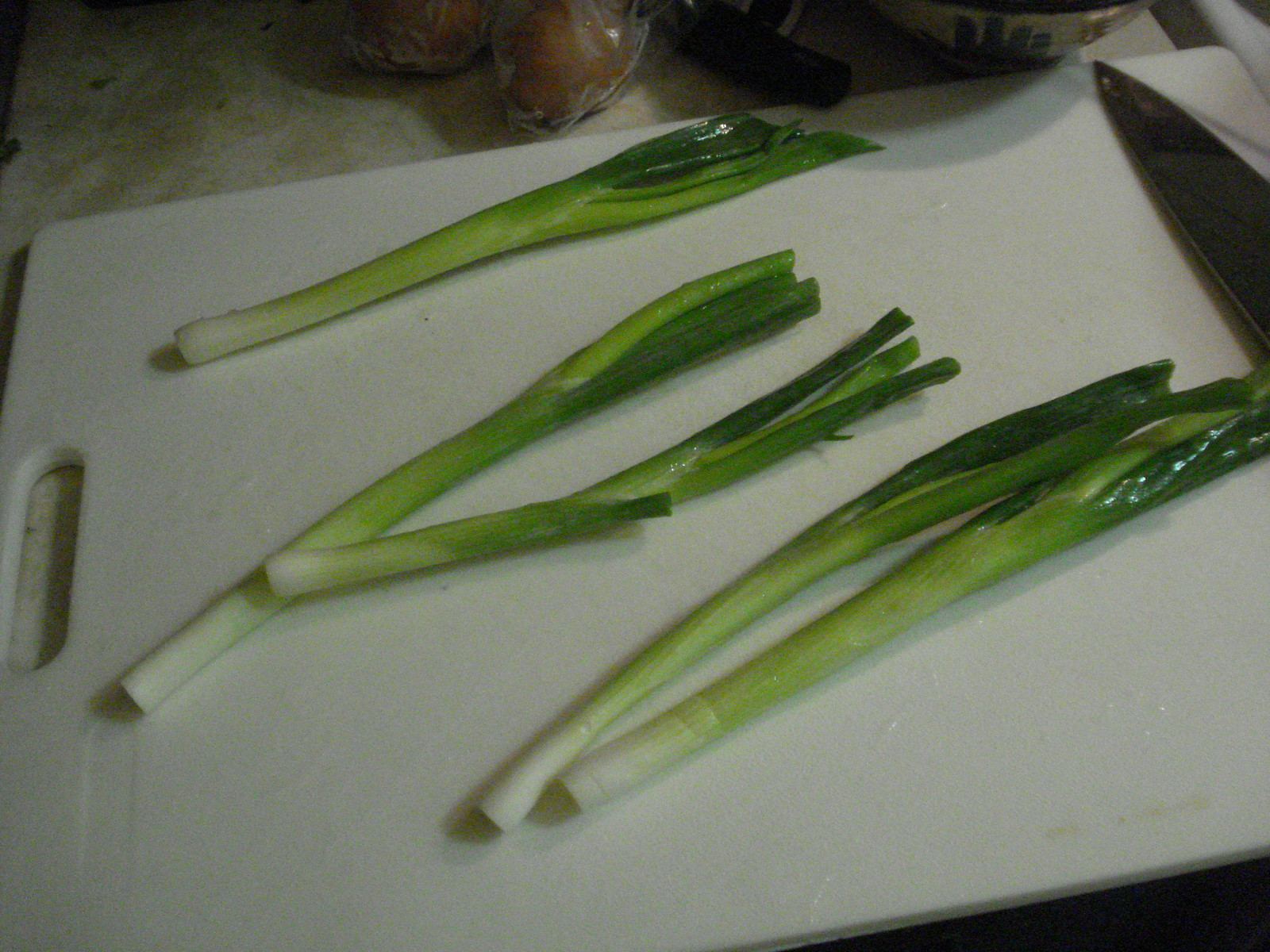The photograph depicts a white plastic cutting board with a handle cutout on the left side, resting on a white marbled countertop. On the cutting board lie five stalks of celery, each transitioning from white at the base to dark green at the leafy tips. The celery stalks appear wet and fresh. In the upper right corner of the image, the blade of a large metal knife slightly intrudes into the frame, though its handle and the bottom portion of the blade are cut off. The background is cluttered with indistinct items, including brown oval shapes in a plastic bag, which could be either potatoes or eggs, and a partially visible bowl. The photograph is a detailed close-up with no text, people, or animals present.